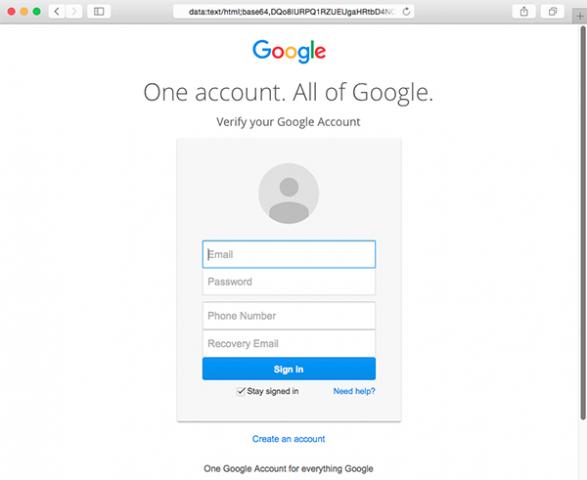The image depicts a Google account verification page displayed on a computer screen. At the top of the page, there is a prominent Google logo. Below the logo, a gray, large-font text reads "One account. All of Google." Underneath this text, a smaller gray font instructs the user to "Verify your Google account."

The main section of the page features a form with fields for the user to enter their email address, password, phone number, and recovery email as part of the sign-in process. There's an option to stay signed in, and for those new to the service, a blue hyperlink at the bottom of the form prompts users to "Create an account."

At the very bottom of the page, a statement in gray text reads "One Google Account for everything Google." The URL of the page is unusually complex and formatted as "data.txt.html;base64,DQ," followed by a series of numbers and letters which seem nonsensical and unrelated to typical web addresses.

In summary, this image captures the standard Google account login screen with a peculiar URL format.